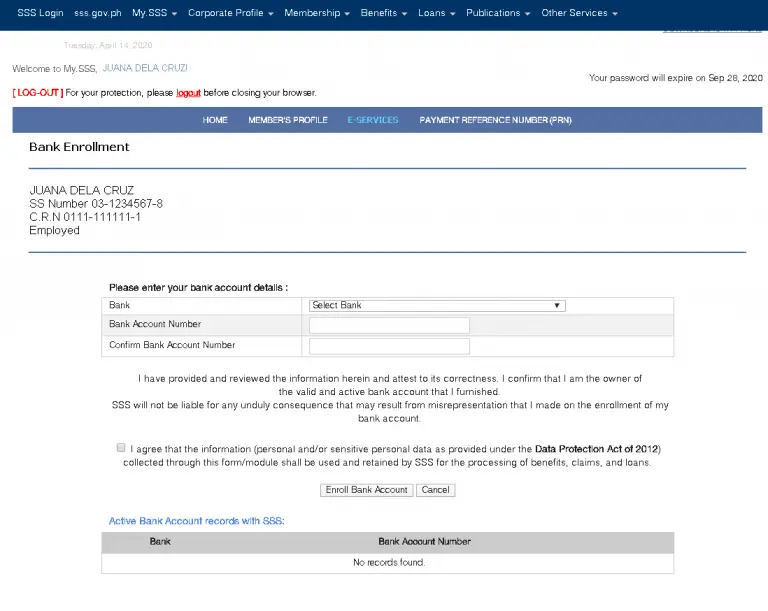The image depicts a user interface of the SSS (Social Security System) website, specifically the section where a user, who is logged in, is prompted to enter their information. At the top of the screen, in a navy blue rectangle, there are various navigation tabs labeled as follows: "ssslogin," "sss.gov.ph," "My SSS," "Corporate Profile," "Membership," "Benefits," "Loans," "Publications," and "Other Services." Each tab, starting from "sss.gov.ph," features a downward-facing triangle, indicating the presence of a dropdown menu for additional options.

Directly below the navigation bar, the website displays the current date, "Tuesday, April 14th, 2020," in a light gray font. Beneath this date, a prominent welcome message reads, "WELCOME TO MY SSS, AWANA DE LA CRUZ," in all capital letters.

Towards the left of the screen, there is a section for "Bank Enrollment." This area appears to be designed for users to enter and confirm their bank account details, including fields for the bank account number and its confirmation.